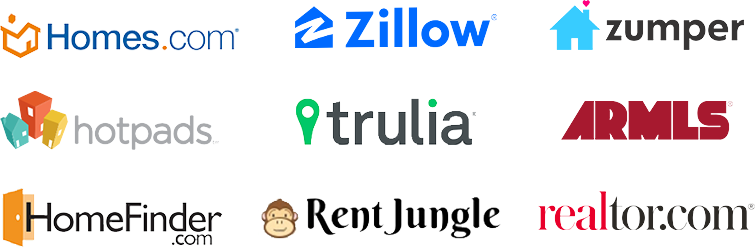The image showcases a neatly arranged display of various real estate service labels, each accompanied by a distinctive icon. 

1. **Homes.com**: Represented by a simple house icon.
2. **Zillow**: Features a diagonally-placed "Z" within a house shape.
3. **Zumper**: Illustrated with a blue house topped by a small red heart.
4. **HotPads**: Depicts a complex image of a house alongside two tall buildings, the one on the right resembling a townhouse.
5. **Trulia**: Characterized by a green accent on the side.
6. **ARMLS**: Shown simply with the block letters "ARMLS".
7. **HomeFinder.com**: Identified by an icon of an open door.
8. **RentJungle**: Features the playful image of a monkey.
9. **Realtor.com**: The word “real” is highlighted in red, with the rest of the text in black. 

Each icon adds a unique visual element that enhances the brand identity of the respective real estate services.